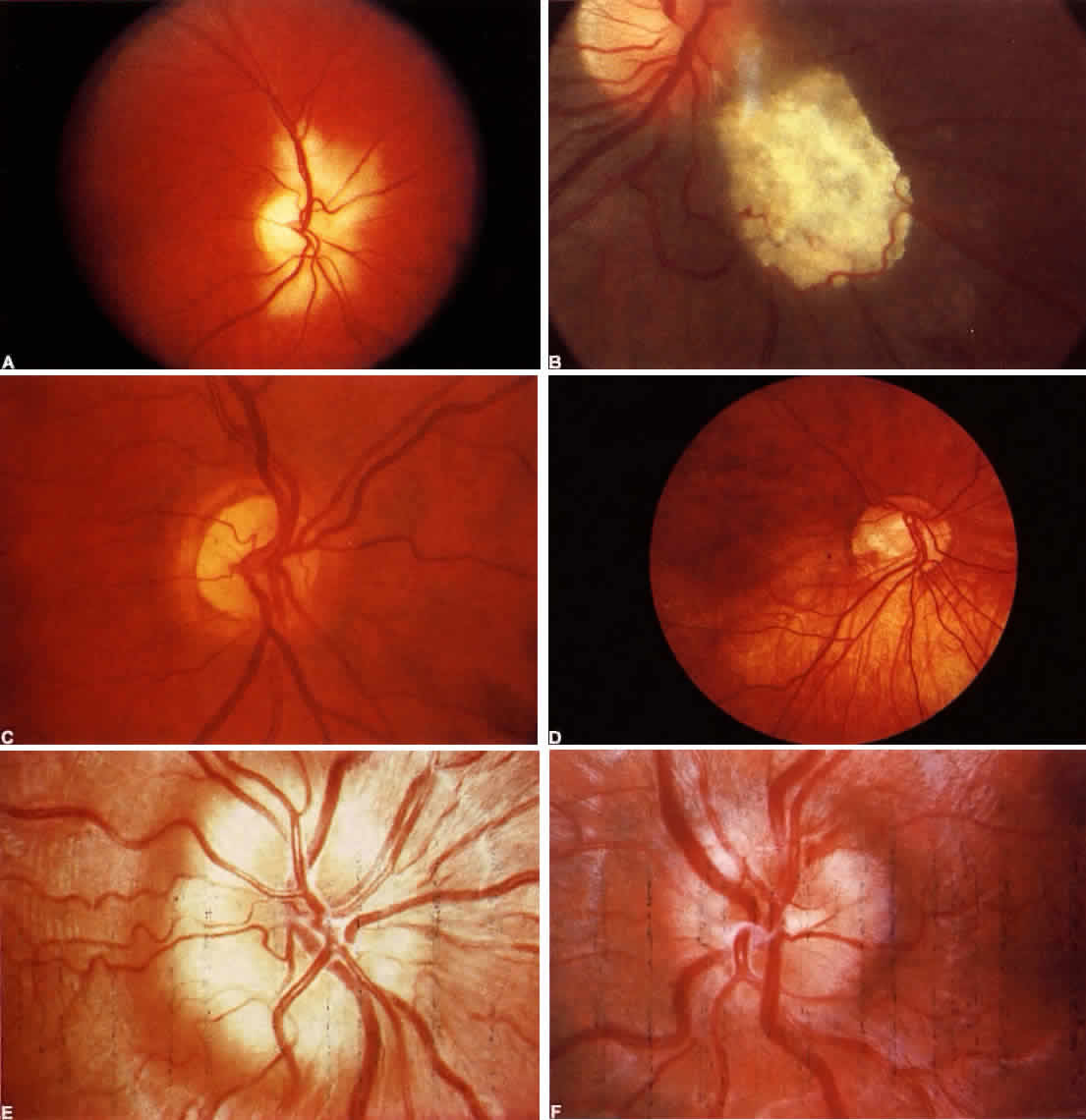This intricate collage comprises six distinct images labeled A, B, C, D, E, and F, arranged in three rows and two columns, each with text in white color positioned in the bottom left corner. The images depict the round structure of an eye, showcasing the pupil, cornea, and prominently visible red veins that create a web-like pattern throughout. With a mix of close-up shots and different perspectives, the eye's textures are highlighted, bringing out hues of red, yellow, and white in the pupil and cornea. Two of the images stand against a stark black background, emphasizing the vivid colors and intricate details. This cohesive series, possibly captured by a medical professional, intricately illustrates the eye's anatomy, focusing on the blood vessels and the varied textures seen within each photograph.